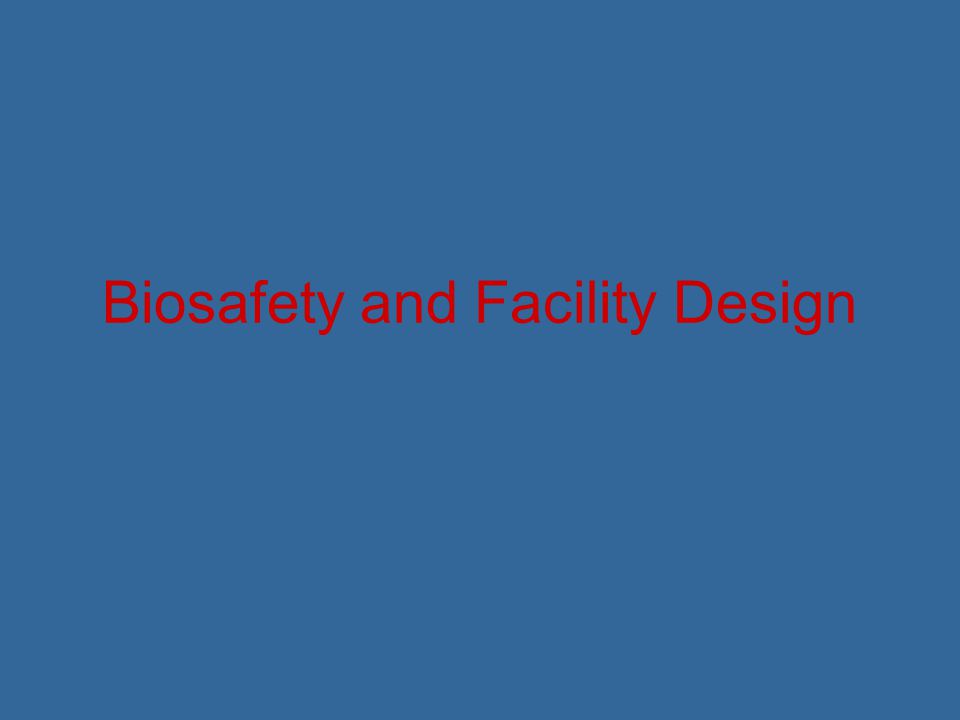The image features a simple, educational slide with a slate blue, rectangular background that has a slightly grayish, old-fashioned hue. In the center of the slide, raised slightly from the middle, is the phrase "Biosafety and Facility Design" written in a bold, red font. The deep red text, set against the dusky blue background, creates a visually striking effect that almost seems to make the words pop out of the image. Each significant word begins with a capital letter, while "and" is in lowercase. Subtle JPEG artifacting adds some minor distortion around the text, showing slight variations in the blue and red colors.